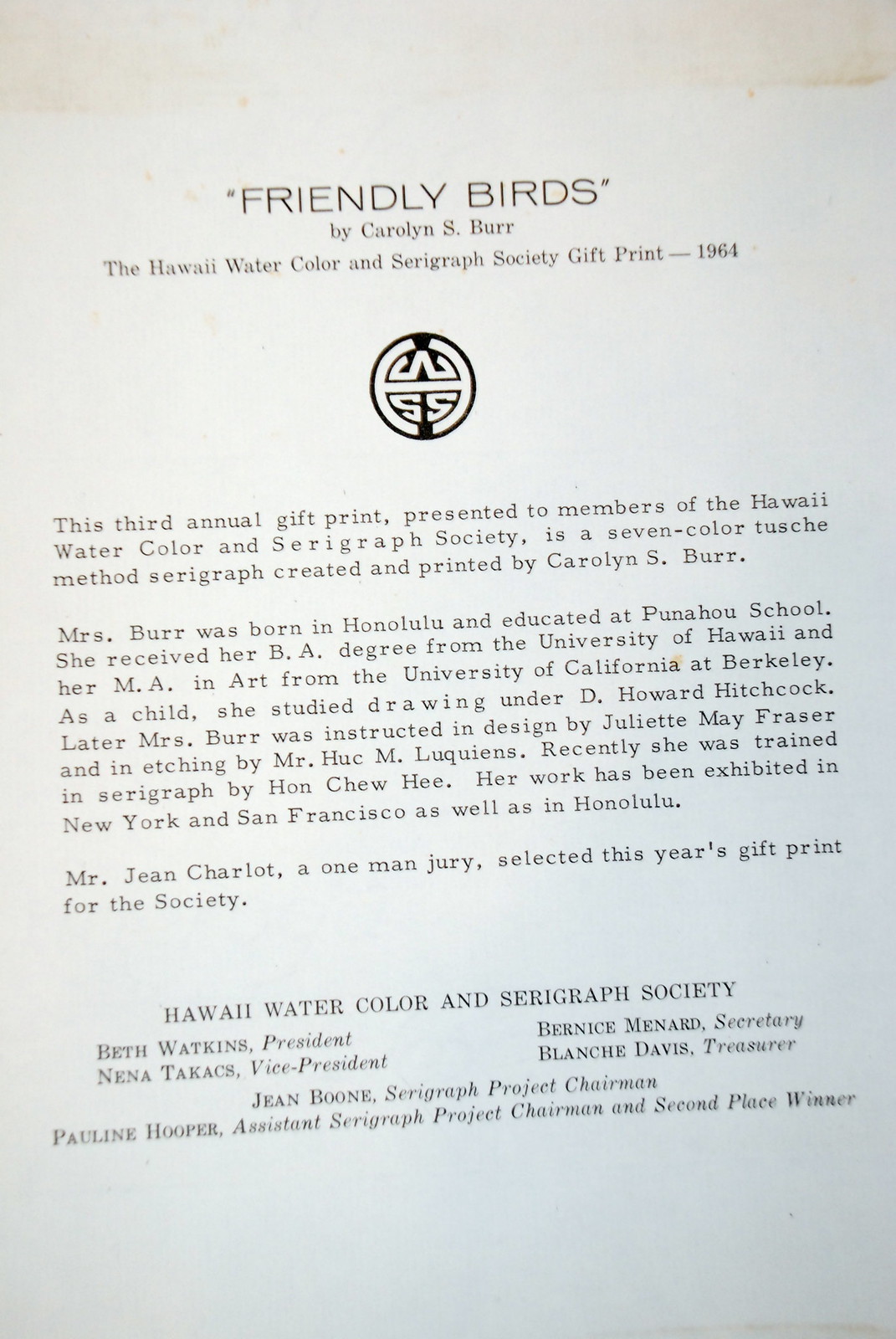The image depicts a detailed, white printed page titled "Friendly Birds" by Carolyn S. Burr. Centered at the top, the title is highlighted in the largest text. Below it reads: "The Hawaii Watercolor and Serigraph Society Gift Print 1964." Underneath, separated by a small insignia of the society, the text continues: "This third annual gift print, presented to members of the Hawaii Watercolor and Serigraph Society, is a seven-color touche method serigraph created and printed by Carolyn S. Burr."

The next section offers a brief memorial to Carolyn S. Burr, noting that she was born in Honolulu, educated at Punahou School, and earned her BA degree from the University of Hawaii, followed by an MA in arts from the University of California at Berkeley. Her early art education included studying drawing under D. Howard Hitchcock and design tutelage from Juliet May Fraser, with later training in etching by Mr. Huck M. Lukens and in serigraphy by Han Shu He. Burr's works have been showcased in prestigious exhibitions in New York, San Francisco, and Honolulu.

The document further notes that Mr. Gene Charlotte, serving as a one-man jury, selected this year's society gift print. At the bottom, it lists the society's overseeing members, including President Beth Watkins, Vice President Nina Takas, Secretary Bernice Menard, Treasurer Blaich Davis, Serigraph Project Chairman Jean Boone, and Assistant Serigraph Project Chairman Pauline Hooper, who is also noted as the second-place winner.